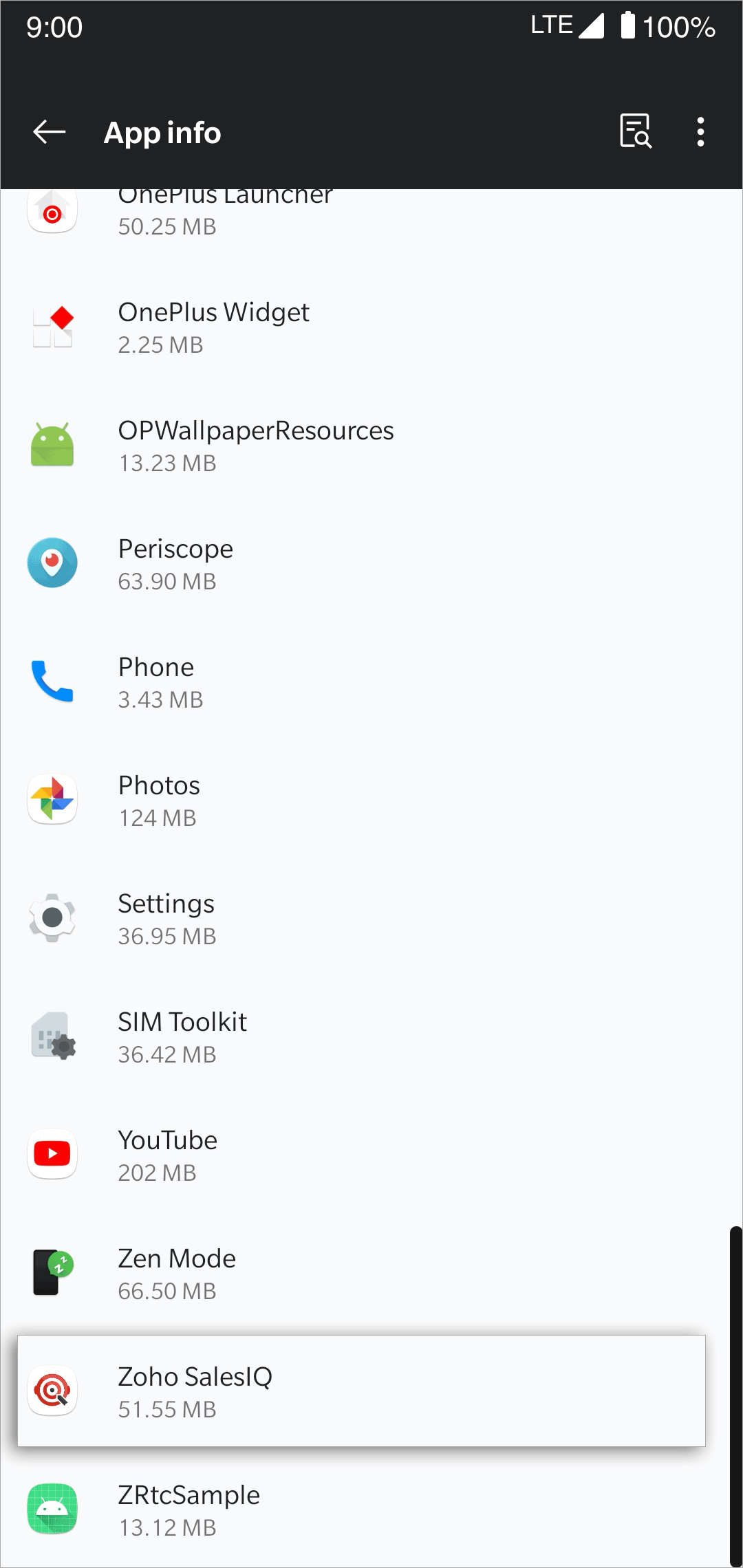The screenshot depicts a smartphone interface with a detailed status bar and a list of applications. The top header is black, featuring the current time displayed as "9:00" in white on the left side, although it does not specify AM or PM. On the right side, it shows "LTE" in white capital letters, accompanied by icons for a full wireless network signal and a fully charged battery at 100%.

Below the header, on the left side, the text "App Info" appears in white against the black background, with a left-pointing arrow symbol next to it.

The main part of the image has a white background displaying a lengthy list of various apps, with each app's icon positioned on the left side. The list includes, from top to bottom, the following applications: OnePlus Launcher, OnePlus Widget, OP Wallpaper Resources, Periscope, Phone, Photos, Settings, SIM Toolkit, YouTube, Zen Mode, Zoho Sales, and at the very bottom, ZRTC Sample.